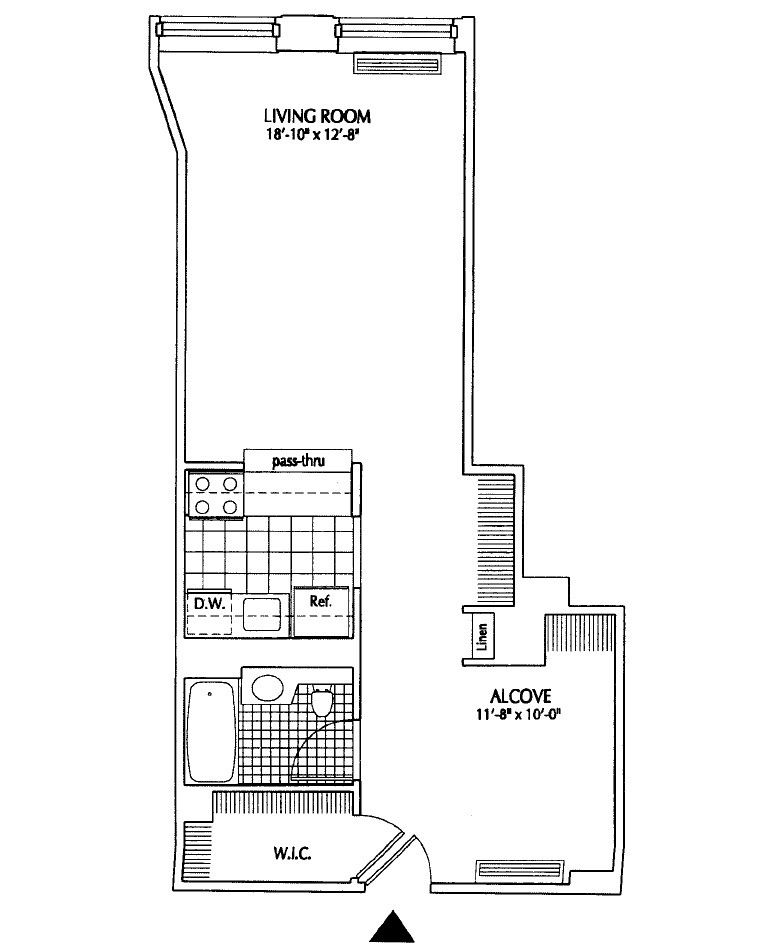This detailed floor plan, illustrated in black ink on a white background, depicts a residential unit. The layout features a long vertical rectangular shape with an extension on the right side, from the center down to the bottom. At the bottom center of the plan, a black triangle points upward towards two lines and a semicircle, symbolizing the main entrance.

Upon entering, to the left is a small room labeled "WIC" (Walk-In Closet). To the right is a larger square room named "Alcove," measuring 11 feet 8 inches by 10 feet 0 inches. Moving further up the hallway on the left side, there is a bathroom followed by a kitchen. The kitchen's layout includes a stove positioned on the upper left wall and a pass-through window opening into the living room.

Adjacent to the alcove on the right, there's a linen closet. The long hallway continues upward, leading into a spacious living room, which slightly bends to the left at the top. The living room is labeled "Living Room," with dimensions of 18 feet 10 inches by 12 feet 8 inches. A window is centered on the upper wall of the living room, providing natural light to the space.